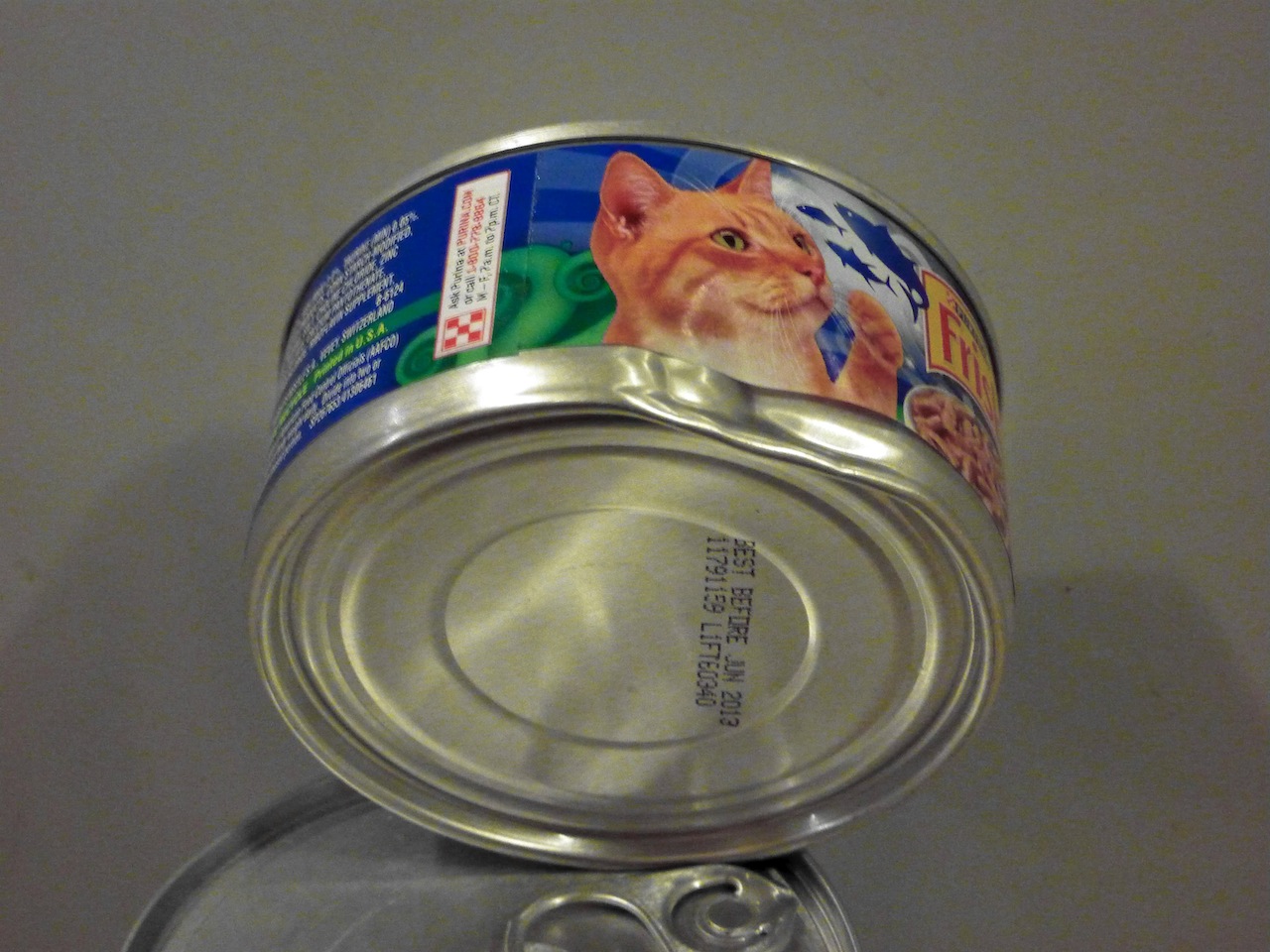A dented can of Friskies cat food, featuring a blue label, lies horizontally atop another can of the same brand. The damaged can prominently displays an orange tabby cat with raised paw, positioned against a background with a swimming shark. Adjacent to the cat is a partially visible customer service phone number and an ingredient list, confirming the product is made in the USA. The Friskies logo is situated above an image of cat food to the right of the feline illustration.